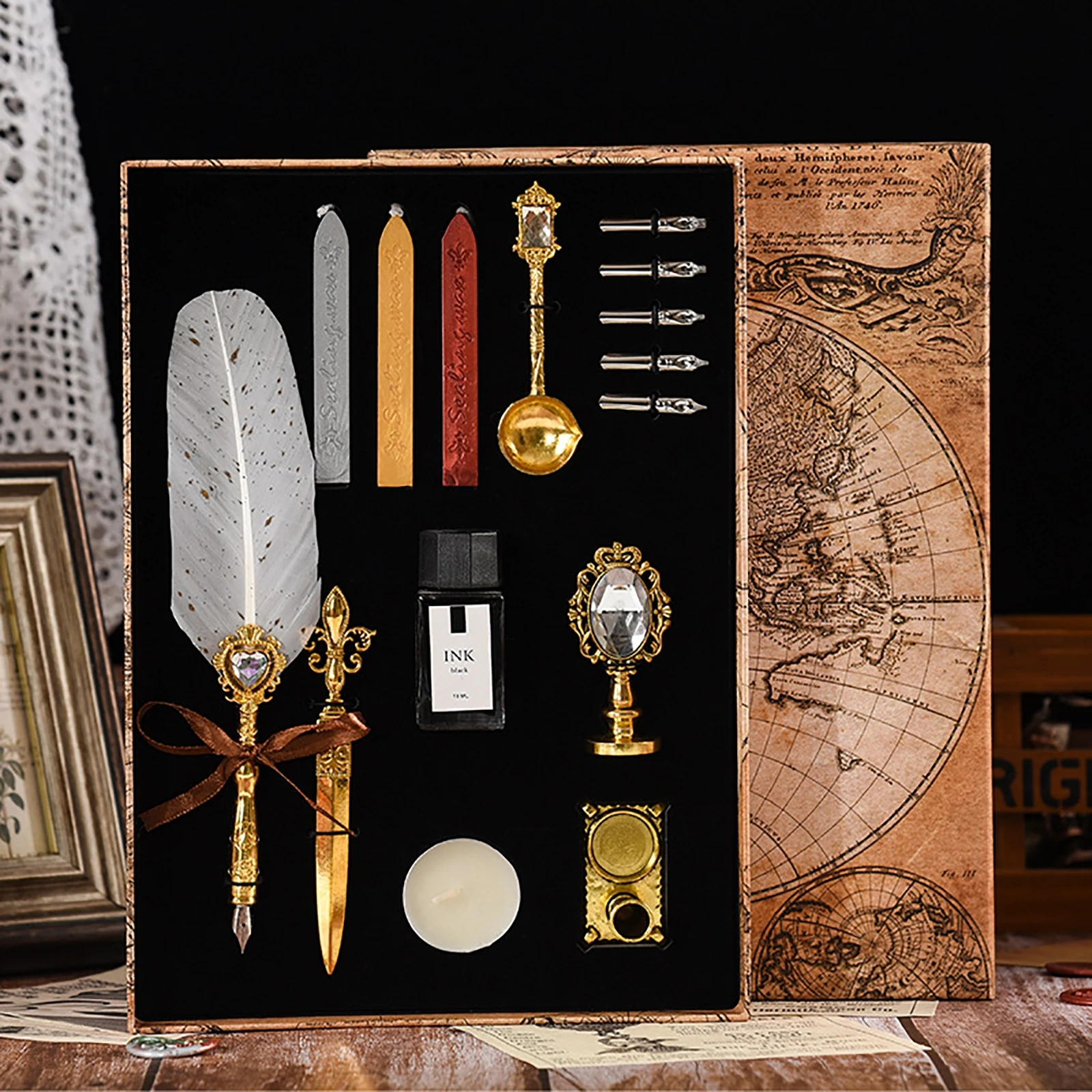The photograph showcases an elegantly arranged feather quill pen set, prominently displayed on a wooden table against a dark backdrop. Central to the display is a bottle labeled "Ink," surrounded by an array of writing tools, including five pen nibs and a large feather quill pen with a white feather. The set also features a spoon containing wax in shades of gray, yellow, and red, intended for sealing. In the bottom-left corner, two luxurious gold pens are tied together with a red ribbon. The assortment also includes a small tray for the ink and a landscape picture or globe image, along with an indistinct photo in a frame and a lacy white blanket. The color palette of the image includes bronze, gold, white, and red, contributing to the set’s vintage and refined aesthetic.